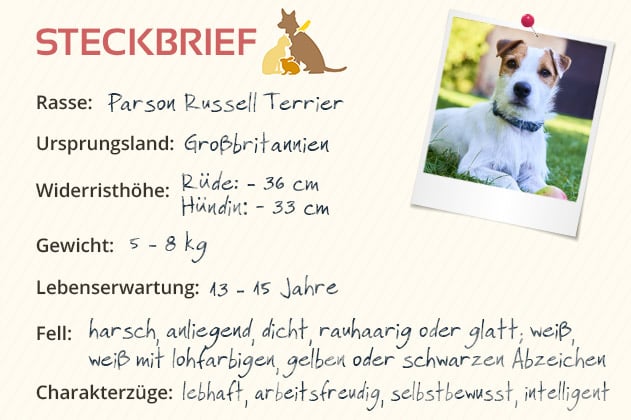The image is a detailed informational card about a Parson Russell Terrier. The card, about 4x6 in size and made of light beige cardstock with a slight texture, has "Steckbrief" in red letters at the top left, which translates from German to "profile." Below this title is a graphic featuring a dog, cat, and bunny, suggesting it might be from a veterinary clinic or pet adoption agency. On the right side, a photo of the dog—a white terrier with a blue collar, brown fur around its eyes, and brown floppy ears—is pinned to the card with a simulated thumbtack.

The card contains various non-English, specifically German, categories and details about the dog. The breed is listed as "Rasse: Parson Russell Terrier," and its origin is noted as "Erbsprungslind: Großbritannien" (Great Britain). Additional measurements and characteristics include the dog's height ("Rüde 36 cm, Hündin 33 cm"), weight ("Gewicht: 5-8 kg"), and age ("Alter: 13-15 Jahre"). The card also includes information on the dog’s temperament and traits, briefly mentioned in English as intelligent.